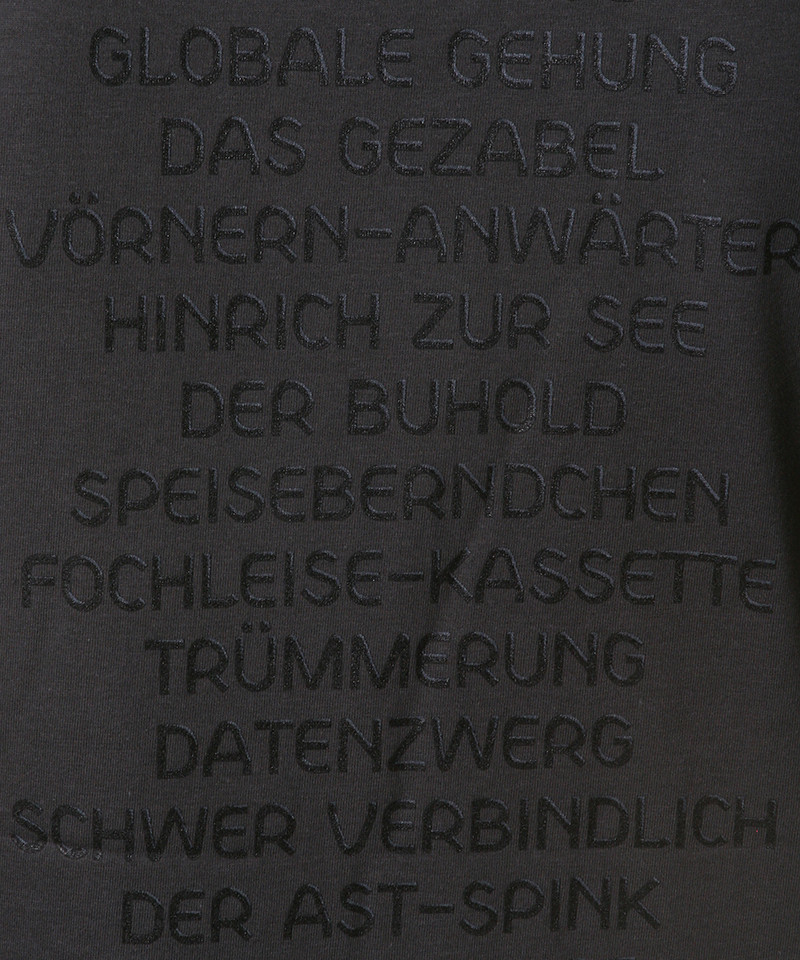This image features an intricate engraving on a dark gray, sandy rock-like surface. The inscriptions are meticulously carved in a clean, precise, sans-serif font and are all in uppercase letters, showcasing a grayish hue against the gray background. The text appears to be in German and reads, starting from the top:

"GLOBALE GEHUNG DAS GEZABEL VÖRN-ANWARTER HINRICH ZUR SEEDER BUHOLD SPEISEBERNDCHEN FOHLEISE-KASSETTE TRUMMERUNG DATENZWERG SCHWER VERBINDLICH DER AST-SPINK".